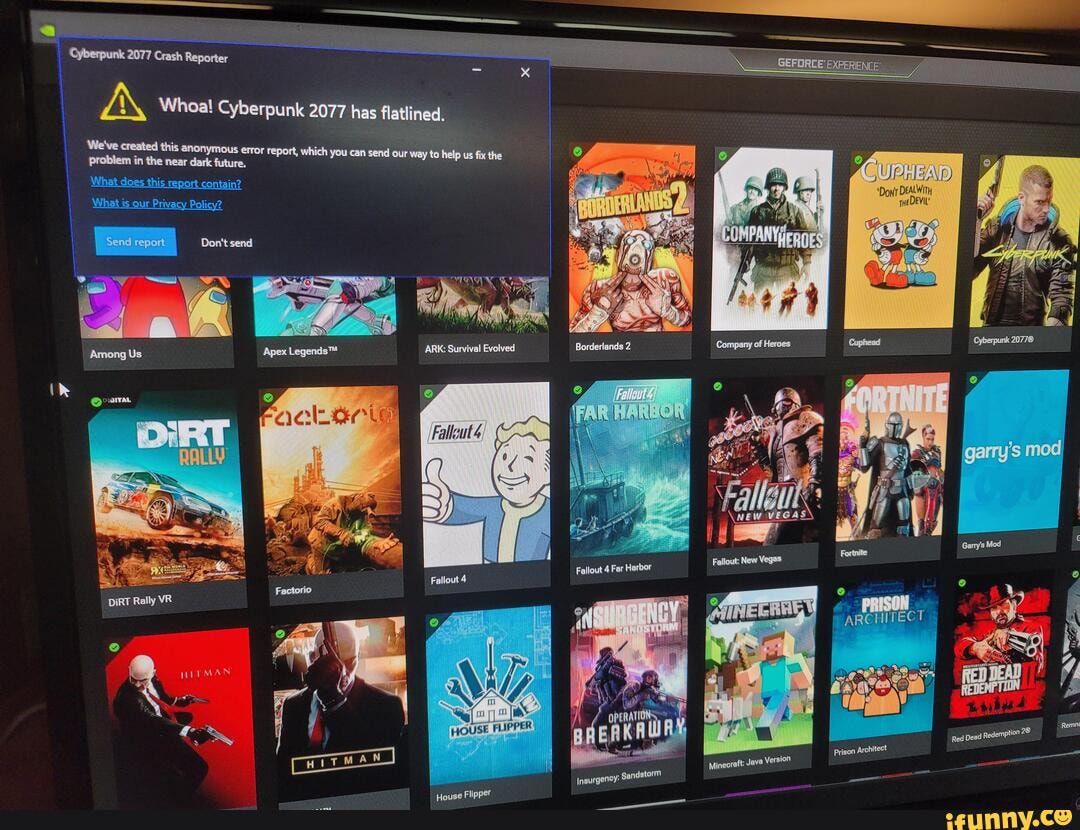A screenshot of a gaming platform's library interface showcasing the notification for the completion of "Cyberpunk 2077" download. The screen displays an array of game covers, including popular titles like "Fallout," "Cuphead," and "Dirt Rally," among others. The vibrant and varied game icons create a visually engaging collection, reflecting a diverse gaming repertoire. Each game cover is meticulously designed, adding a colorful and dynamic element to the interface.